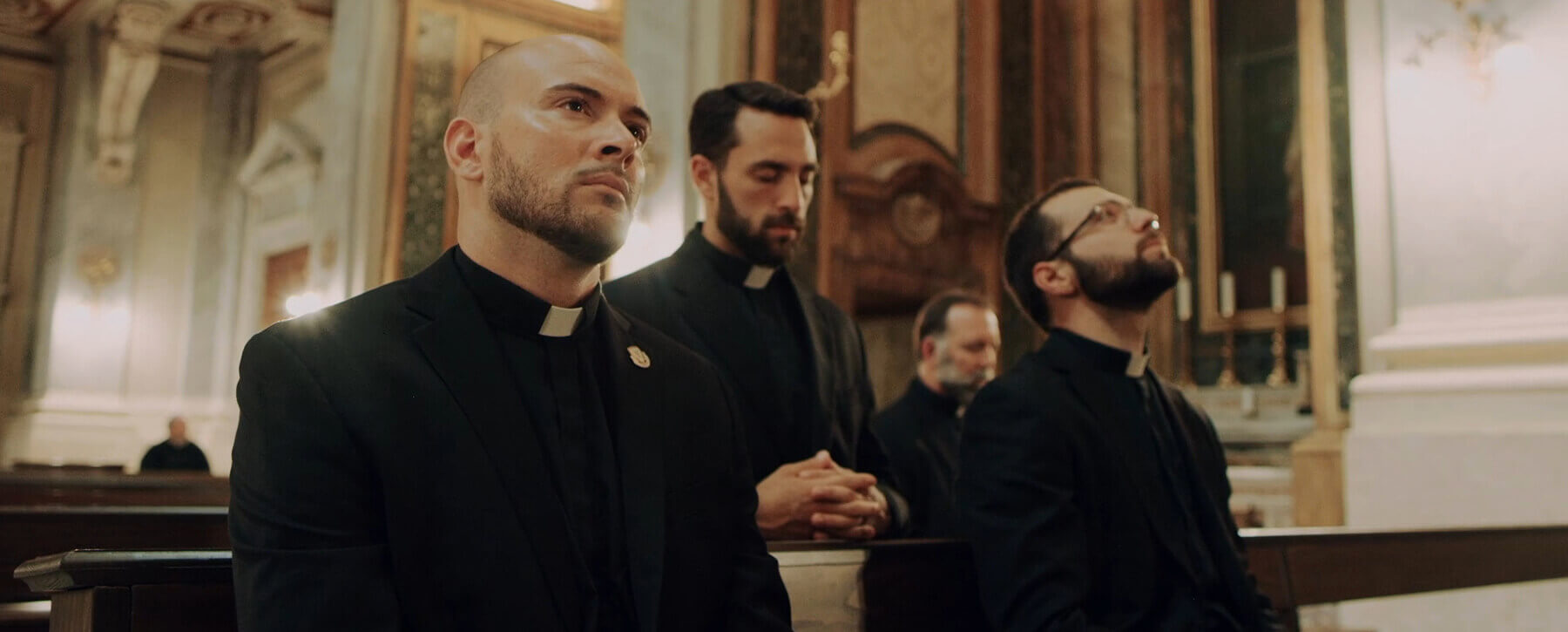The full-color photograph, taken indoors in a well-lit church with white walls and beautiful ceiling arches, features four clergymen prominently in the foreground. All four priests, ranging in age from their 30s to 40s, have beards and are dressed in traditional black cassocks with white collars. The bald priest on the left, who has a low-cut beard and mustache, appears to have a pin on his robe. Next to him, sharing the same pew, is a priest with dark hair, a thick mustache and beard, and glasses, holding his hands clasped together in prayer. Behind them is another priest with dark hair and a full beard and mustache, but without glasses. On the far right, a priest with a graying beard, dark hair, and a mustache looks up, seemingly in deep thought or meditation. In the background, a fifth figure dressed in black can be seen, though it's unclear if he is also a clergyman. The setting, adorned with arches and warm artificial lighting, reinforces the serene and solemn atmosphere typical of a church. Three candles are visible near the center right, enhancing the spiritual ambiance of the scene.